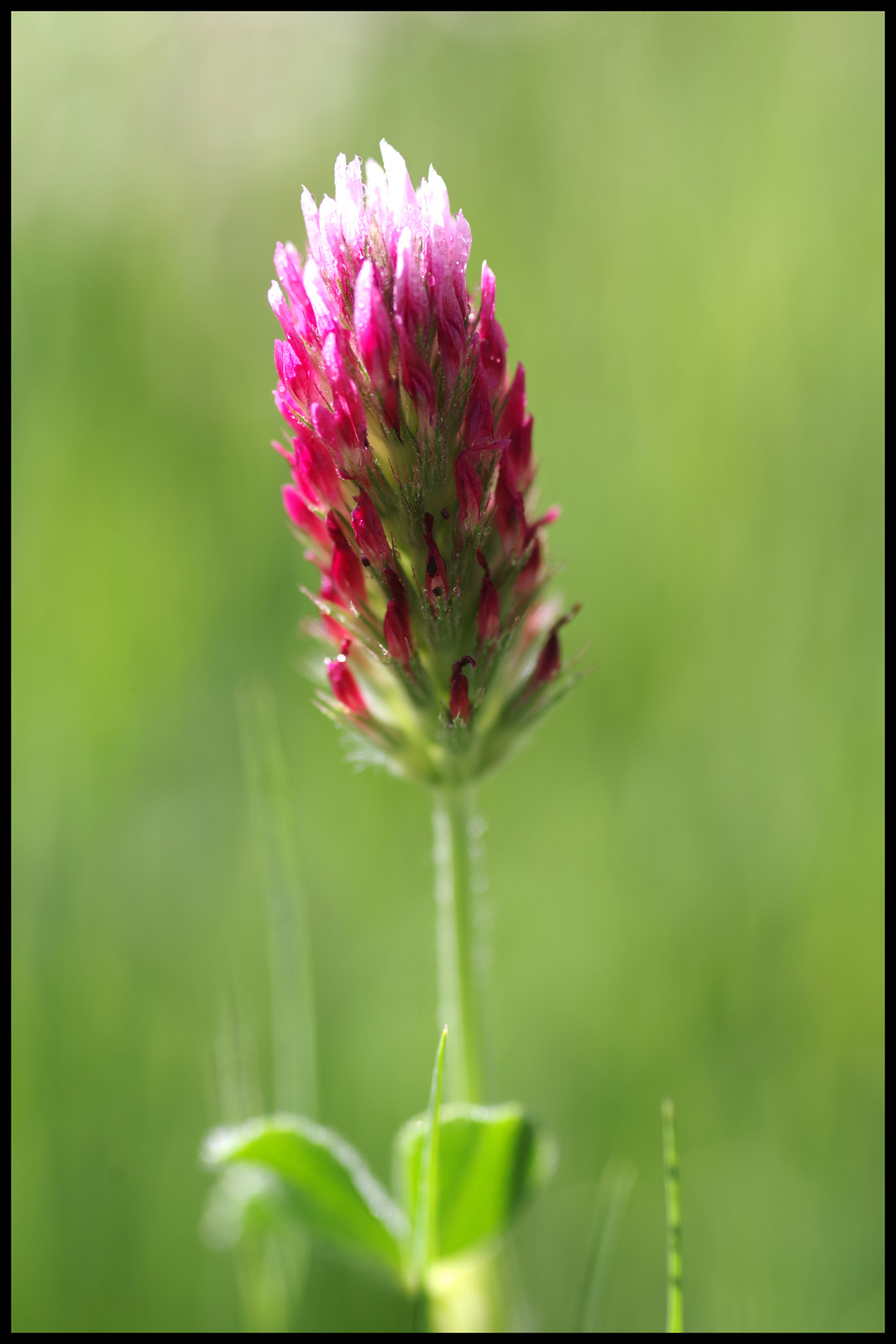This photograph captures an extreme close-up of a striking pink flower with a blurred, lime green backdrop, rendering the overall composition simple yet mesmerizing. The flower has not fully bloomed, and its cluster of petals, which resemble the seed clusters of a raspberry or a rabbit's foot, are primarily pink with lighter white tips. These lighter tips might be due to sunlight or the flower's development stage. The flower has a green stem with some green elements at its base, contributing to the overall aesthetic. The use of a narrow depth of field ensures that the background is entirely out of focus, giving the image a mystical, almost painted quality. The lack of any identifying text or labels enhances its potential for art gallery displays or online showcases.